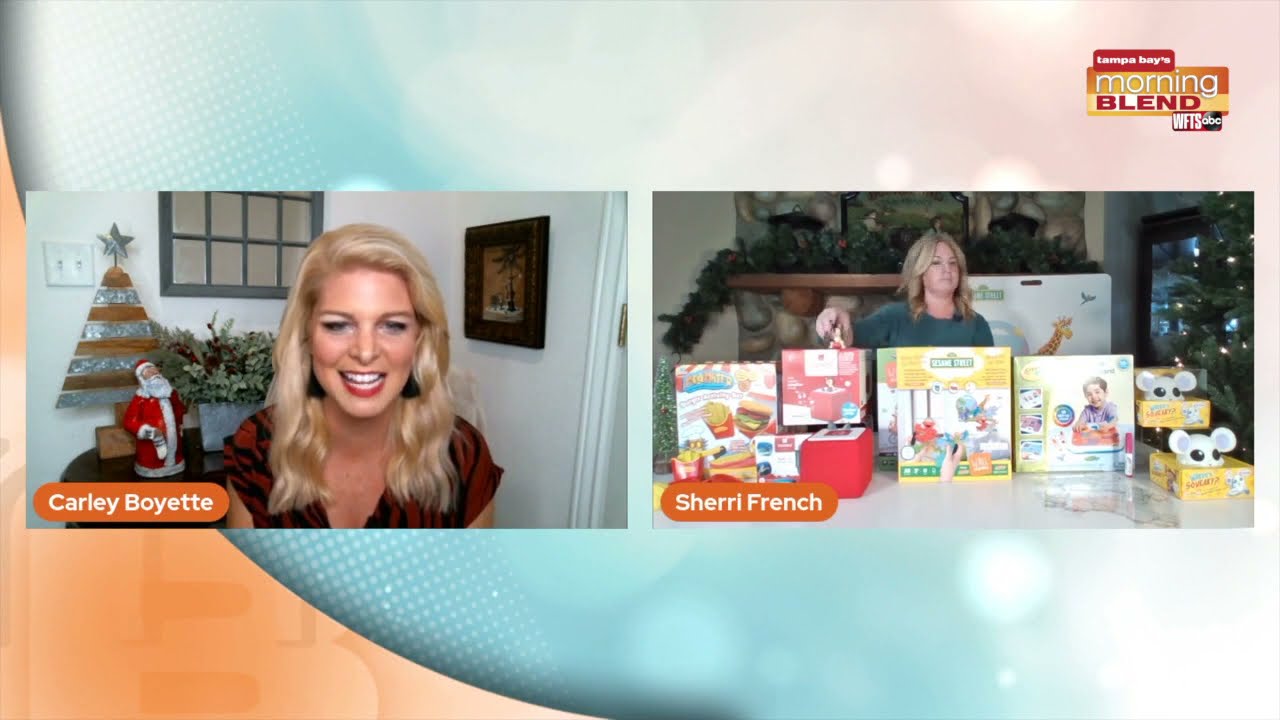The image is composed of side-by-side screenshots from the Morning Blend TV show, set against a festive blue, orange, and light pink gradient background. The backdrop features a small 'Tampa Bay's Morning Blend WFTS ABC' logo in orange, red, and white on the upper right.

On the left, we see Carly Boyette's segment. She is seated in a corner of her home with white walls adorned with colorful Christmas decorations, including a Santa Claus, a small Christmas tree, holly, and berry arrangements. A painted window pane and a framed picture also embellish the background. Carly, with her blonde hair, is smiling warmly at the camera, wearing an orange and black animal print blouse.

To the right, Sherry French stands behind a table filled with boxes that appear to be children's toys. Her background is equally festive, showcasing a Christmas tree to her right and garlands. Sherry, also blonde, is engaged in her segment, perhaps discussing or showcasing the toys displayed in front of her.

Both sections of the image are clearly labeled with the names "Carly Boyette" and "Sherry French" in the lower left corners of their respective frames.